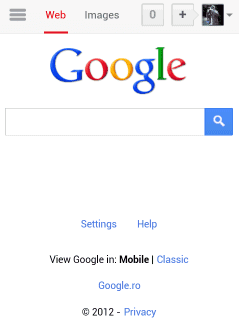This image portrays a Google search interface with notable elements. Centered at the top is the Google logo, featuring its iconic blue, red, yellow, and green colors. Directly below the logo, an empty search bar invites user input, accompanied by the familiar Google search button. To the left of the search bar, three horizontal lines denote a menu or navigation icon, while to the right, "WEB" is highlighted in red, with "IMAGES" following it. A square containing a zero and another with a plus sign are aligned to the side. Beneath the search bar, blue links for "Settings" and "Help" are displayed. Further down, a suggestion to "View Google in Mobile" is followed by the class identifier "google.ro" and the year "2012." At the bottom, there is a clickable "Privacy" link in blue. The top right corner features a small avatar icon resembling a picture of a man, likely indicating a user profile option.